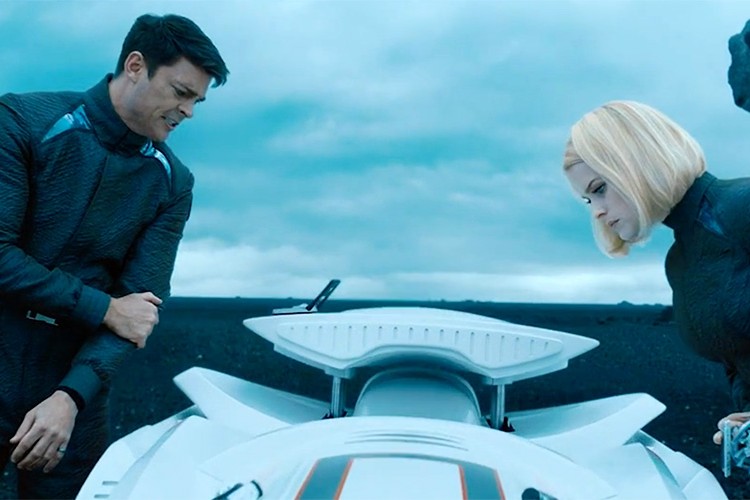In this image, a man and a woman are closely examining a sleek, white vehicle with blue and light orange accents, likely a race car or futuristic craft. The man, positioned on the left, has short black hair and is dressed in a black suit. His arm is crossed, holding his elbow, and he gazes intently downward. He is white, handsome, and appears slightly older. The woman, on the right, has jaw-length blonde hair and also wears a similar black suit, suggesting they might be drivers or characters in a sci-fi setting. She appears younger and stares neutrally at the vehicle. The background features a blurred expanse of sky and ground, reinforcing the scene's high-tech ambiance.